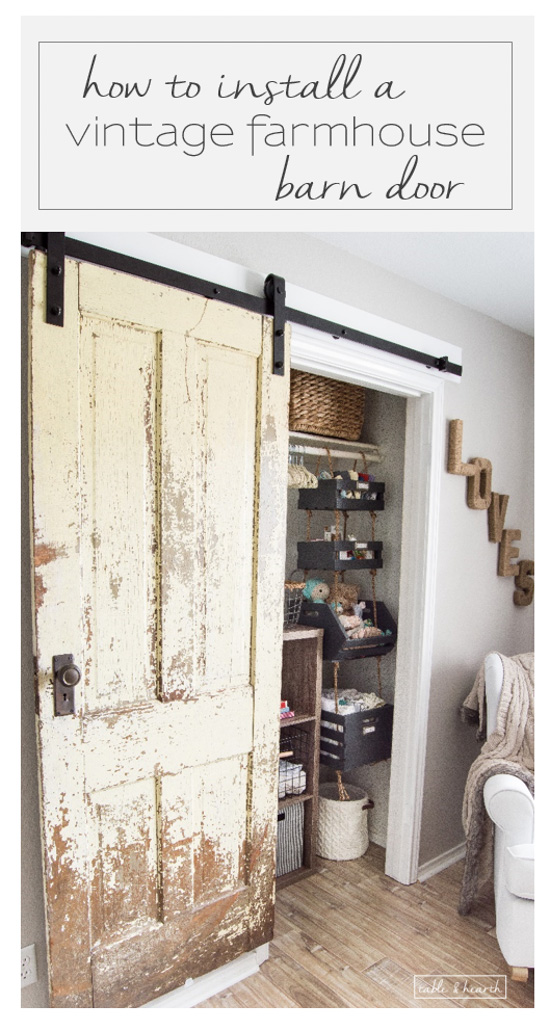The photograph captures a charming juxtaposition of old and new within a modern home. The focal point is a small, vintage-style door mounted on black sliders to function as a closet door. This barn door is heavily distressed, with white paint chipped away significantly, especially at the bottom, revealing the old wood underneath. A dark iron doorknob accentuates its antique appeal. Inside the closet, modern elements like hanging black baskets filled with stuffed animals and clothing can be seen suspended from a rod, along with a glimpse of a wooden shelf. The closet is framed by white borders, and the entire setup is nestled against very light gray walls and light brown wooden flooring. Adjacent to the closet, wooden letters spell out "L-O-V-E-S" in a descending diagonal, suggesting a personalized touch. Above the entire scene, a long rectangular frame features black text that instructs on "how to install a vintage farmhouse barn door," with part of the text in cursive and part in print, enhancing the blend of old-fashioned charm and contemporary decor. Additionally, a cozy white padded chair with an afghan draped over it hints at the homey atmosphere of the living room where this stylish blend of old and new is showcased.